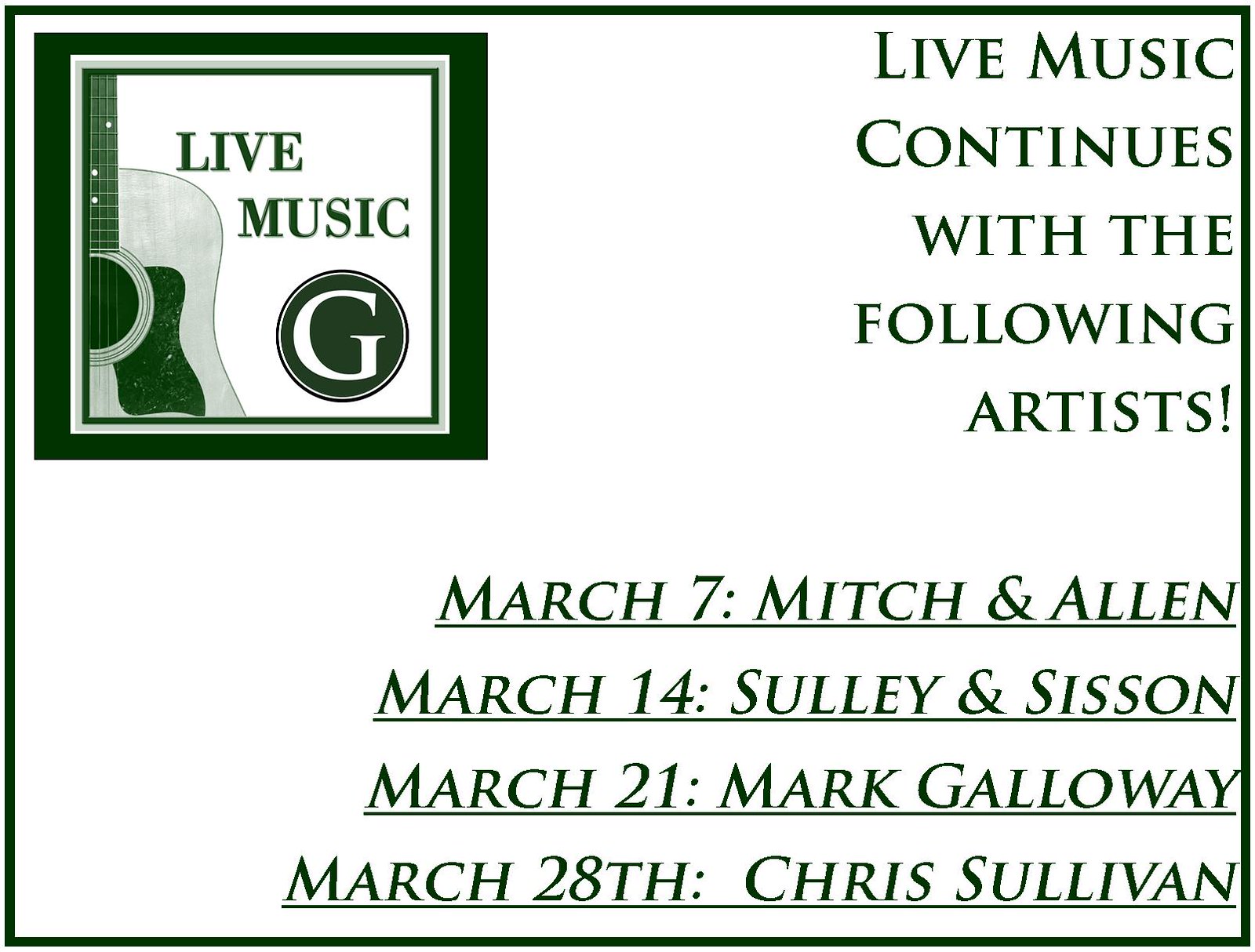This is a detailed flyer for an upcoming live music festival. The background is white, and prominently in the upper left corner, there is an image of a wooden guitar, partially visible and featuring shades of light and dark green. Written in green, it says "Live Music" beside the guitar. Adjacent to this, there's a dark circle containing a white capital "G." The text reads "Live music continues with the following artists:" followed by an exclamation point. Presented in a large, easy-to-read green font, the schedule lists the performances: "March 7: Mitch and Alan," "March 14: Sully and Sisson," "March 21: Mark Galloway," and "March 28: Chris Sullivan." Each date and artist name is underlined, ensuring the event details are clear and visually organized.